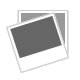In this detailed photographic image, a hand is seen holding up an intricately carved wooden structure against a predominantly white background. The structure, resembling an antique wooden protractor without a central pencil, is propped up by a hand whose four fingers are visible, with the small finger being the most prominent. The wooden object features two long, tapering legs connected about a third of the way up from the base, adorned with identical crisscross and diamond-shaped carvings that suggest tribal or geometric patterns. 

The top of the structure presents a circular, cog-like feature with protruding wooden bits, akin to a dial for adjustment. The face of this circular part resembles a cuckoo clock, adding an element of nostalgic craftsmanship to the piece. The entire surface is etched with meticulous, hand-carved details, making it a captivating piece of wooden art. The combination of angular patterns along the legs and the wheel-like design at the top highlights the artistry and precision involved in creating this beautiful wooden sculpture, which is elegantly displayed by the hand propping it up.